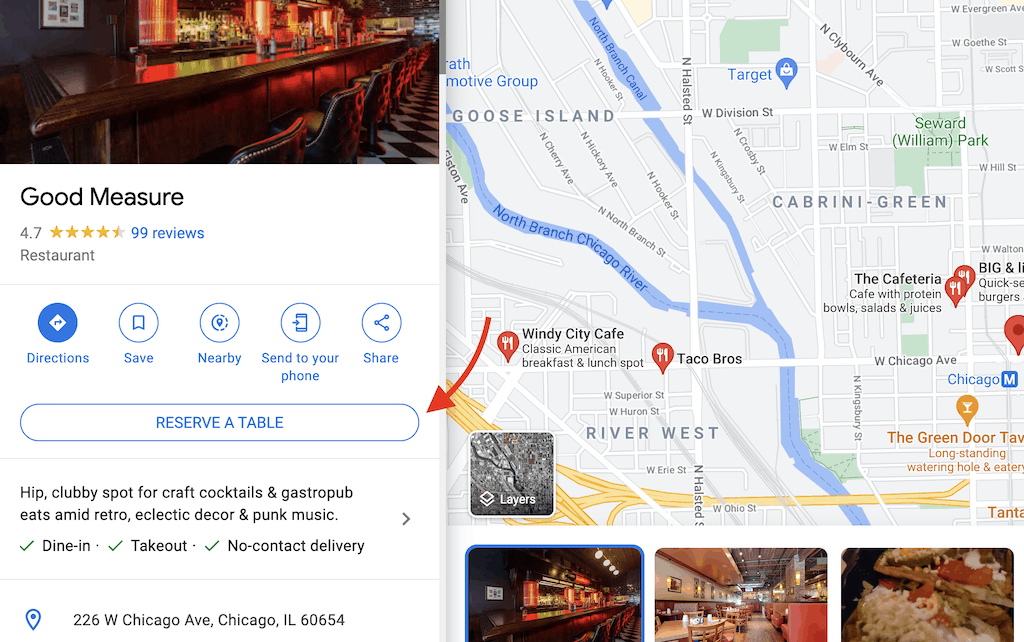This image features the landing page of the restaurant, Good Measure. In the top-left corner, there is a photograph showing the bar area with seating arrangements. Just below this image, the name "Good Measure" is prominently displayed, alongside a rating of 4.7 stars based on 99 reviews. 

To the right, you find a directional map highlighting areas in Chicago, such as Goose Island and Cabrini Green, including landmarks like the Green Door Tavern. Good Measure is pinpointed on Chicago Avenue with an option to "Get Directions." A red arrow points to the "Reserve a Table" button, indicating easy reservations access.

Below the map, there are additional images depicting the bar and some of the restaurant's food offerings. On the left-hand side, just beneath the "Reserve a Table" option, a description reads: "Hip clubby spot for craft cocktails and gastro pub eats amid retro eclectic decor and punk music." The restaurant's address is listed as 226 West Chicago Avenue.